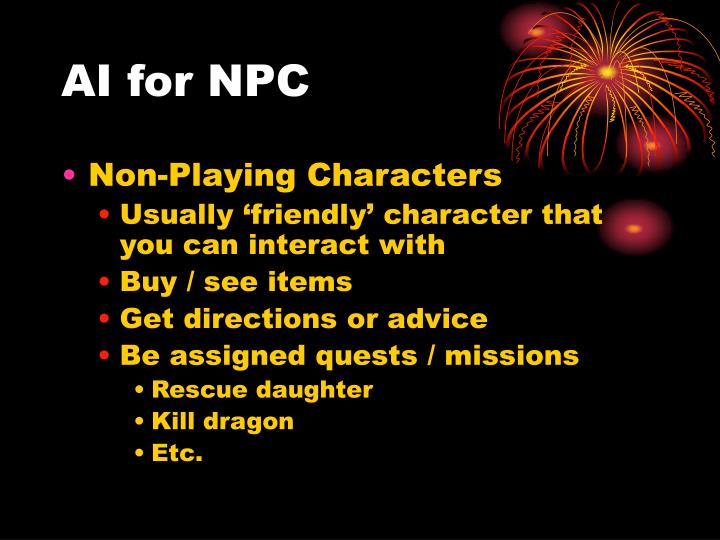The image is a nearly square, card-like presentation featuring text and decorative elements on a dark, black background, reminiscent of a PowerPoint slide. At the very top, "AI for NPC" is prominently displayed in uppercase white font. Below this, a detailed list identifies the roles of non-playing characters (NPCs) in video games, including actions like buying/seeing items, getting directions or advice, and being assigned quests or missions such as rescuing a daughter or killing a dragon. The text primarily appears in yellow and white fonts. The upper right corner of the image showcases red and pink fireworks, adding a festive touch to the predominantly informative layout.